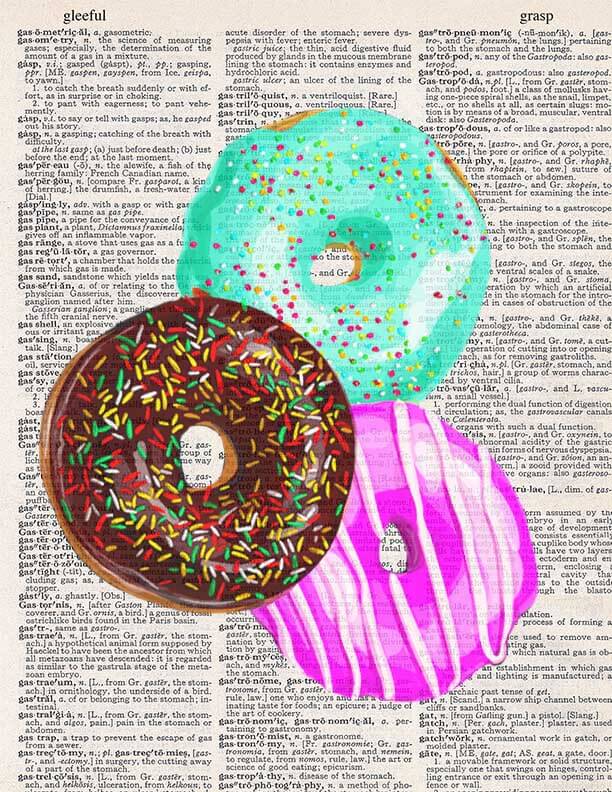This surreal image features a page from an old dictionary, prominently displaying the words "GLEEFUL" and "GRASP" at the top corners. Intriguingly, the main text on this page actually starts with the word "GASOMETRICAL" and concludes with "GATE," encompassing mostly G-A-S words. Overlaid on this dictionary page are three vividly colored doughnuts: a brown chocolate doughnut adorned with red, green, and yellow sprinkles in the forefront, a pink frosted doughnut with additional sprinkles positioned just below it, and a teal frosted doughnut with multicolored sprinkles at the bottom. The combination of the vintage dictionary background and the whimsically colorful doughnuts creates a strikingly surreal juxtaposition.